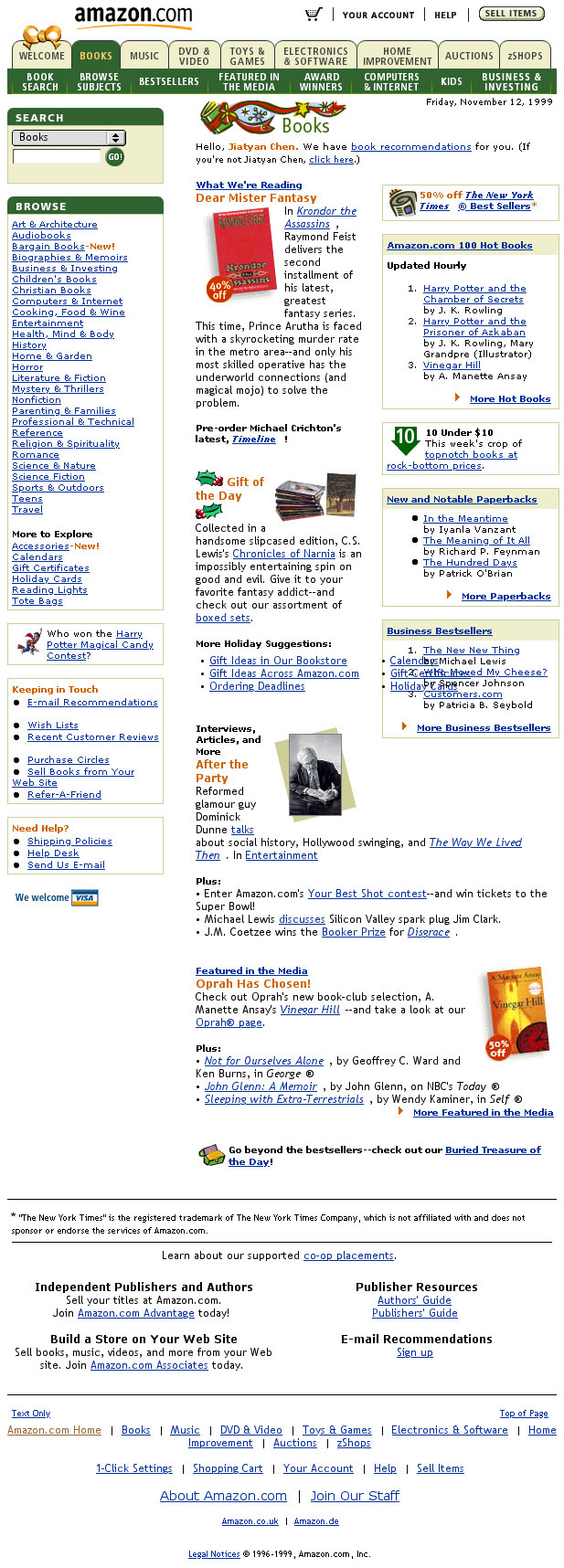This image is a blurry screenshot of an early iteration of the Amazon.com website, identifiable by the Amazon.com logo situated in the top left-hand corner. The logo features "Amazon.com" written in black text, accompanied by a small, curving orange or yellow line beneath it, part of the iconic Amazon smile logo.

The website's interface is predominantly focused on the sale of books, reflecting its original business model. At the top, there are two horizontal navigation bars; the first bar features a series of options in black text against a tan background, while the second bar, located immediately below, has a green background with white text, indicating a different sub-menu.

The page layout is divided into two main columns. On the left-hand side, there are various links designed for browsing different sections of the site, primarily categorized for book shopping. This column hints at the site's early days when Amazon chiefly marketed books.

The right column, occupying the right two-thirds of the page, serves as the main content area. It showcases around four books, each accompanied by a corresponding image and a brief description. Clicking on the links provided with these books would redirect users to a detailed page for more information or to facilitate a purchase. The text throughout the site is mostly in black, used for naming different sections and describing the items available.